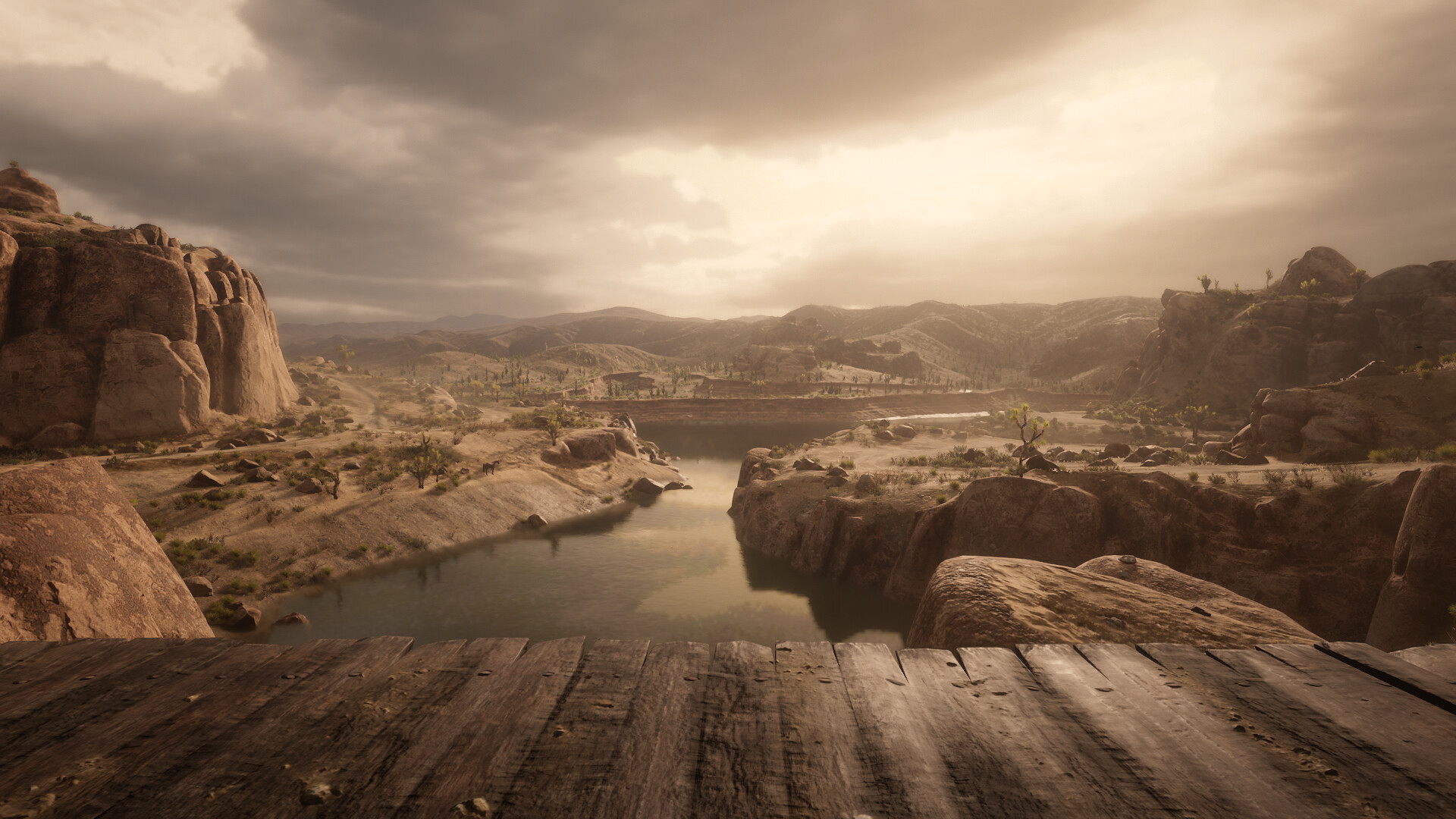The image appears to be a computer-generated depiction of a barren, desert landscape. In the foreground, rough wooden slats, held together by silver nails, form a bridge stretching from the left to the right. This wooden structure, resembling a dock, overlooks a terrain characterized by dusty, brown plains interspersed with sporadic trees and shrubbery. Rocks and rocky outcrops are scattered throughout, leading to a slow-moving body of water that starts from the middle of the scene and winds back towards the horizon. Flanked by brownstone mountains, this waterway seems to continue beneath a distant bridge. The sky is mostly overcast with dark, gray clouds and light brushstrokes of clouds, suggesting an impending dusk. The overall color palette leans towards dark sepia tones, enhancing the desolate beauty of this serene yet stark landscape.